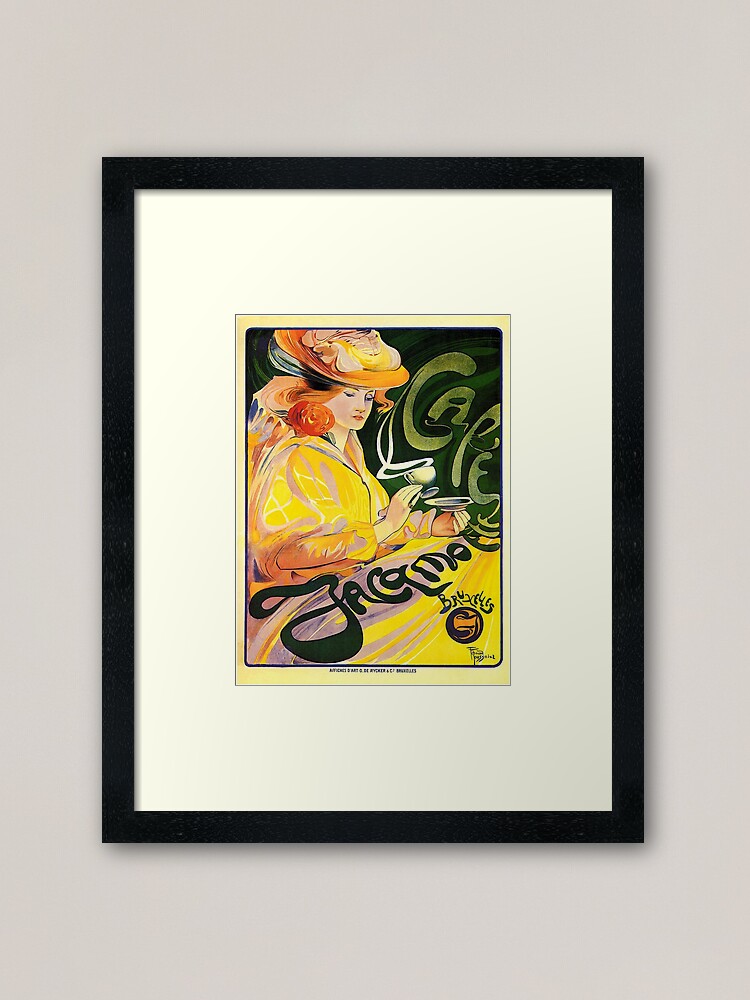The photograph showcases an artwork hanging on a light gray wall. The artwork, encased in a black frame with white matting, appears to be an advertisement poster, possibly French, from the late 1800s to early 1900s. Dominating the scene is a finely dressed woman with red hair, adorned in a long, flowing yellow gown, and a floral hat. Seated elegantly, she holds a steaming cup of coffee in her right hand and a saucer in her left. To her right, the word "CAFE" is prominently displayed in a comical font, followed by more text which appears to read "Tacoma" or "Jackama," though it's partially obscured. Completing the artwork, the bottom right corner features some additional lettering or perhaps the artist's signature, although it is not entirely legible.